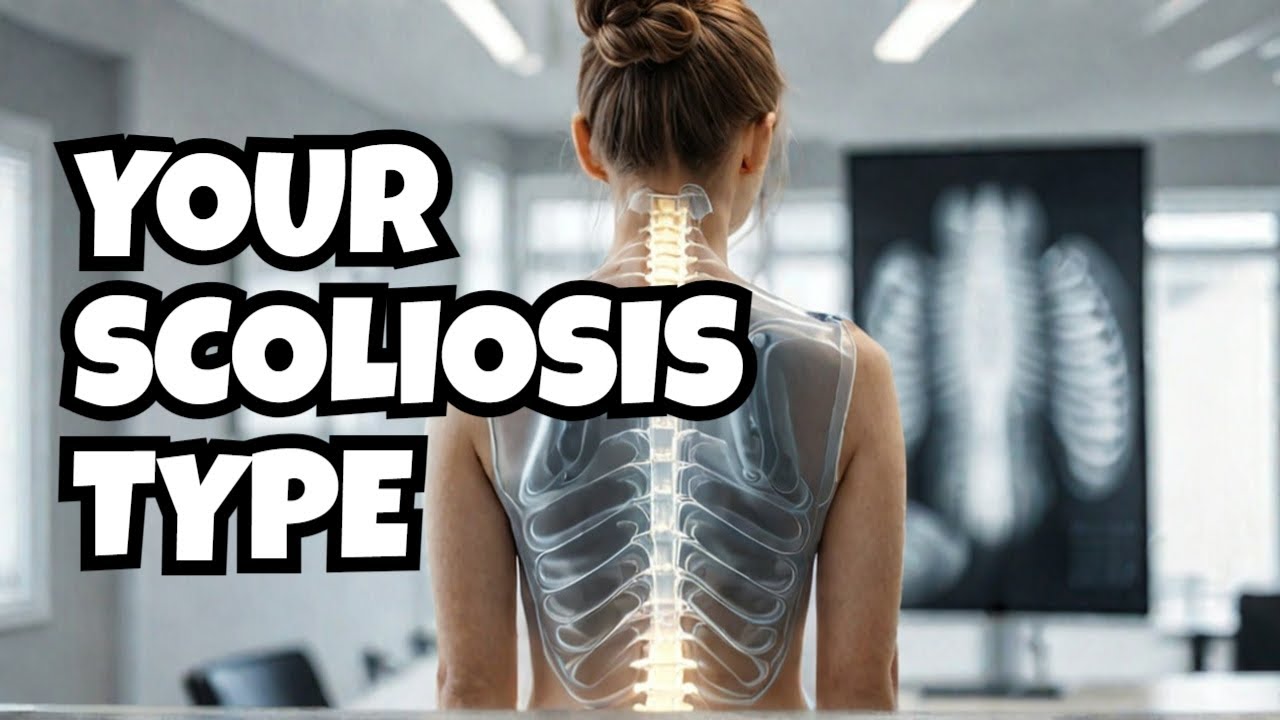This detailed image captures a screenshot potentially from a YouTube video or a medical advertisement about scoliosis. The central figure is a middle-aged, bald man with a greying beard, dressed in a red short-sleeved shirt and blue shorts, sitting barefoot on the floor. His right knee is drawn up with his elbow resting on it, as he points towards an x-ray displayed on the top right. The x-ray reveals a severely curved spine, indicative of scoliosis. Positioned next to the man is a small black table holding a laptop. The background is bright blue with small polka dots. On the left side, there is a yellow square with text in a typewriter font that reads, "Understanding Your Scoliosis from X-Rays." The man appears engaged, speaking directly to the viewer, emphasizing the instructional nature of the content.